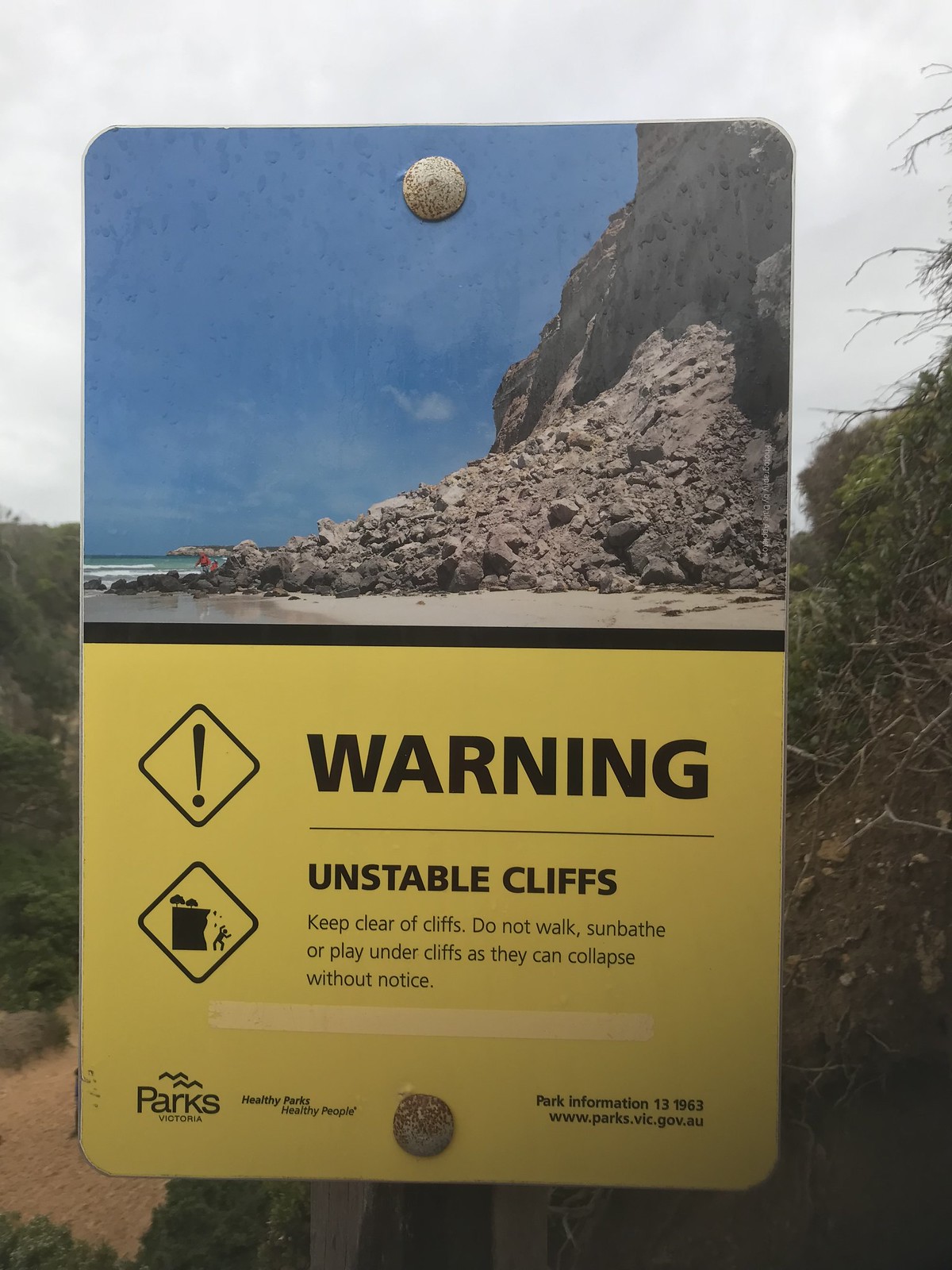This photograph, taken outside on an overcast day, prominently features a metal sign warning about the dangers of unstable cliffs. The sign is divided into two sections: the top part displays a photograph of a cliff wall crumbling into the ocean, while the bottom half, in yellow and red, reads: "Warning! Unstable cliffs. Keep clear of cliffs. Do not walk, sunbathe, or play under cliffs as they can collapse without notice." There are two diamond-shaped warning symbols, one with an exclamation mark and another depicting a person near a collapsing cliff. Additional text at the bottom includes "safe parks" and a website for further information. 

Behind the sign, the environment features muddy brown waters of a river on the left, flanked by cliff sides. More cliffs and some trees are visible in the background to the right. Above, the sky appears stormy and grey, adding to the ominous atmosphere of the scene.